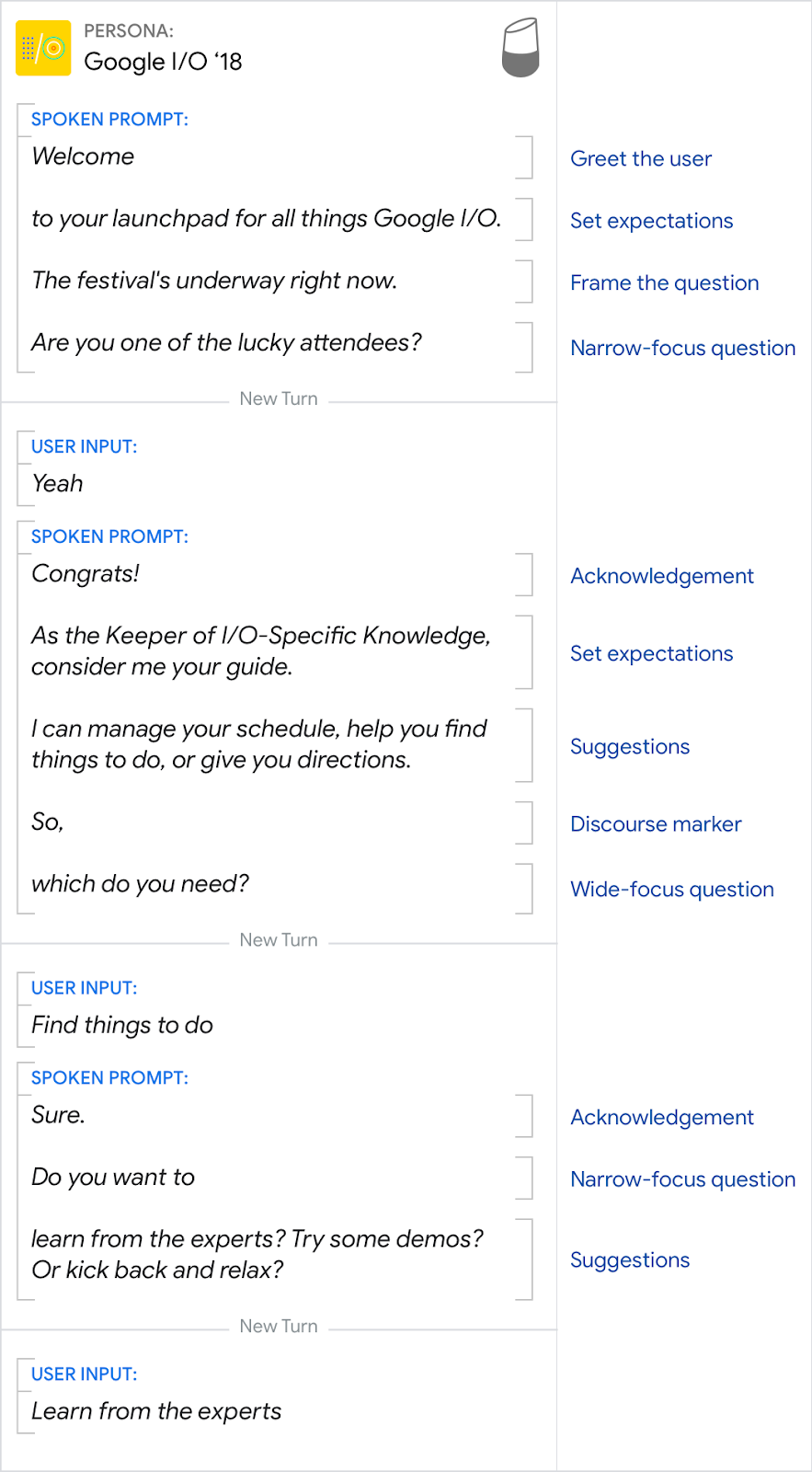The image displays a screen featuring various prompts and details, appearing to be a guide for handling interactions at Google I/O 2018. At the top, the text reads "Persona, Google I/O '18" alongside a yellow icon with blue squares and a green circle.

Under the "Spoken Prompt" section, the text says, "Welcome to your Launchpad for all things Google I/O. The festival's underway right now. Are you one of the lucky attendees?" To the right, there's a message stating "Welcome," with instructions to "Greet the user." Below this greeting, it includes tips to "Set expectations," "Frame the question," and "Ask a narrow focus question."

Under the "New Turn" section, it lists "User Input: yeah." It then transitions to another "Spoken Prompt," where it says, "Congrats," acknowledging the input. The next text advises, "As the keeper of I/O specific knowledge, consider me your guide," categorized as setting expectations.

The guide further states, "I can manage your schedule, help you find things to do, or give you directions," under the "Suggestions" category. Following this, the word "So," is noted as a discourse marker. It then poses the question, "Which do you need?" as a wide-focus question.

The "User Input" section records "Find things to do." In response, the "Spoken Prompt" acknowledges with "Sure," and asks a narrow-focus question, "Do you want to learn from the experts, try some demos, or kick back and relax?" as a suggestion.

Finally, the user input, "Learn from the experts," is listed at the bottom. The overall page has a white background with black and blue text, serving as a comprehensive guide for engaging with various prompts at the event.